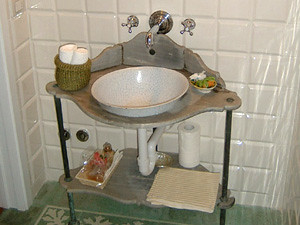This photograph showcases a wall-mounted sink with both the spout and handles affixed to the wall. The water flows into a sleek, bowl-shaped basin with a visible drain at the bottom. The backdrop features a wall adorned with square white tiles, creating a clean and minimalistic look. Below the basin, the floor is covered with green carpeting or a green rug, adding a touch of color to the composition.

Underneath the sink basin, there's a lower shelf that houses essential items. On this shelf, a paper towel and a neatly folded cloth towel are placed, offering functionality and convenience. To the left side of this shelf, a mystery object wrapped in plastic—possibly potpourri—adds an element of intrigue.

Above this shelf, directly beneath the sink, sits a higher shelf. A basket containing a couple of elegantly rolled white washcloths is beautifully displayed for both aesthetic appeal and practical use. To the right of the sink basin, a small bowl—presumably holding soap—completes the scene, though its contents are not entirely clear due to the image's size.

The structural elements of the shelves supporting the sink are gray, contrasting with the black supports that provide sturdy reinforcement. Overall, the image captures a blend of functionality and subtle decor in a bathroom setting.